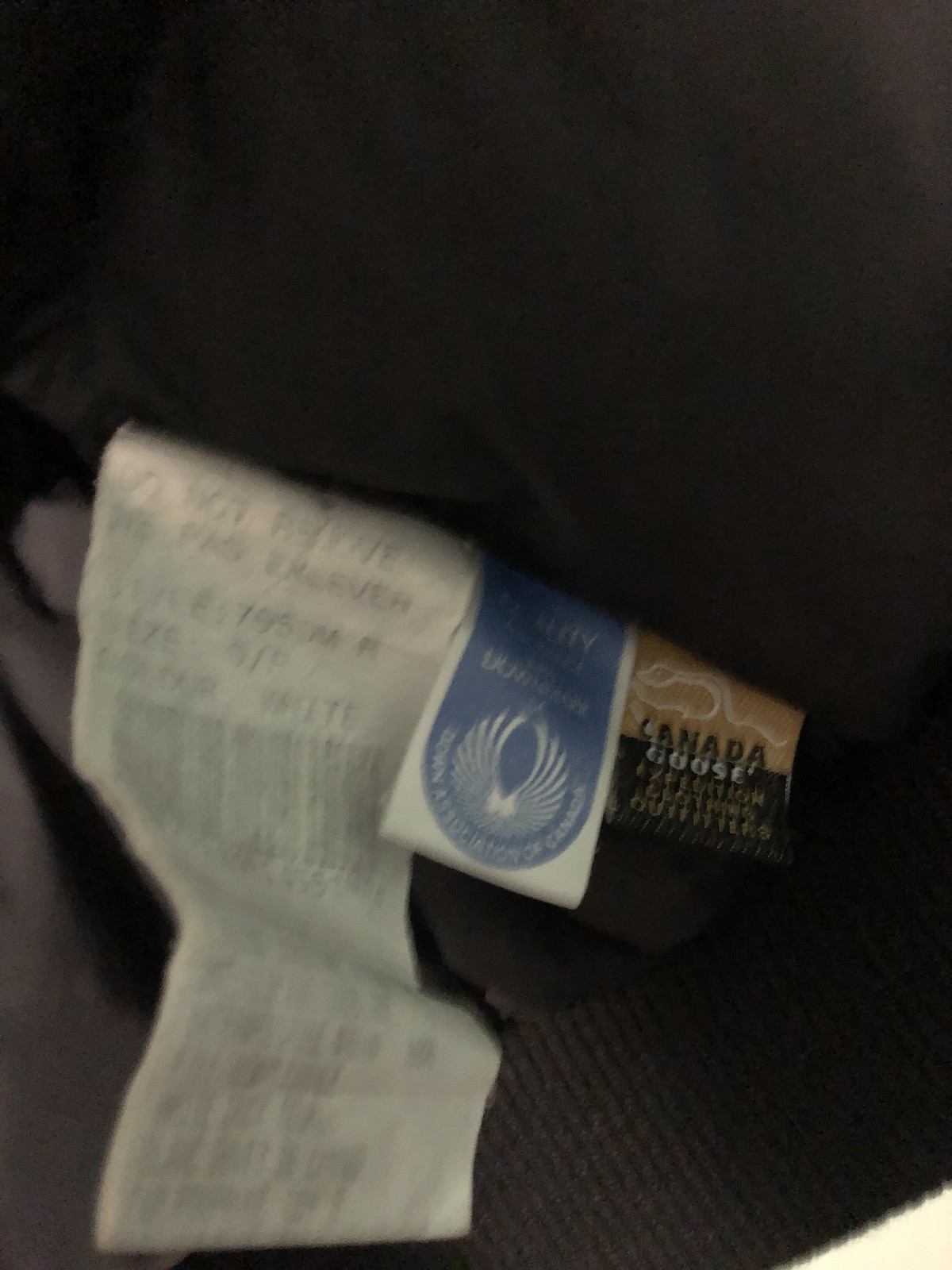The image is quite blurry and out-of-focus, depicting what appears to be various labels attached to a brown, rough-textured sweater. There are three prominent labels. The one on the right reads "Canada Goose Expedition Clothing Outfitters" and is brown and tan in color. The central label is blue and white, displaying the "Down Association of Canada" along with a logo resembling a bird's wings spread upwards. To the left, there's a crumpled, white care label, partially in French, that includes washing instructions, a barcode, and mentions the size as 9 petite. The receipt, found among the labels, is about three inches long but only a couple of inches are visible and it's crumpled in an S shape, making it barely readable. The overall image is set against a dark background, possibly grey or black, with the sweater slightly tilted upwards on the right.